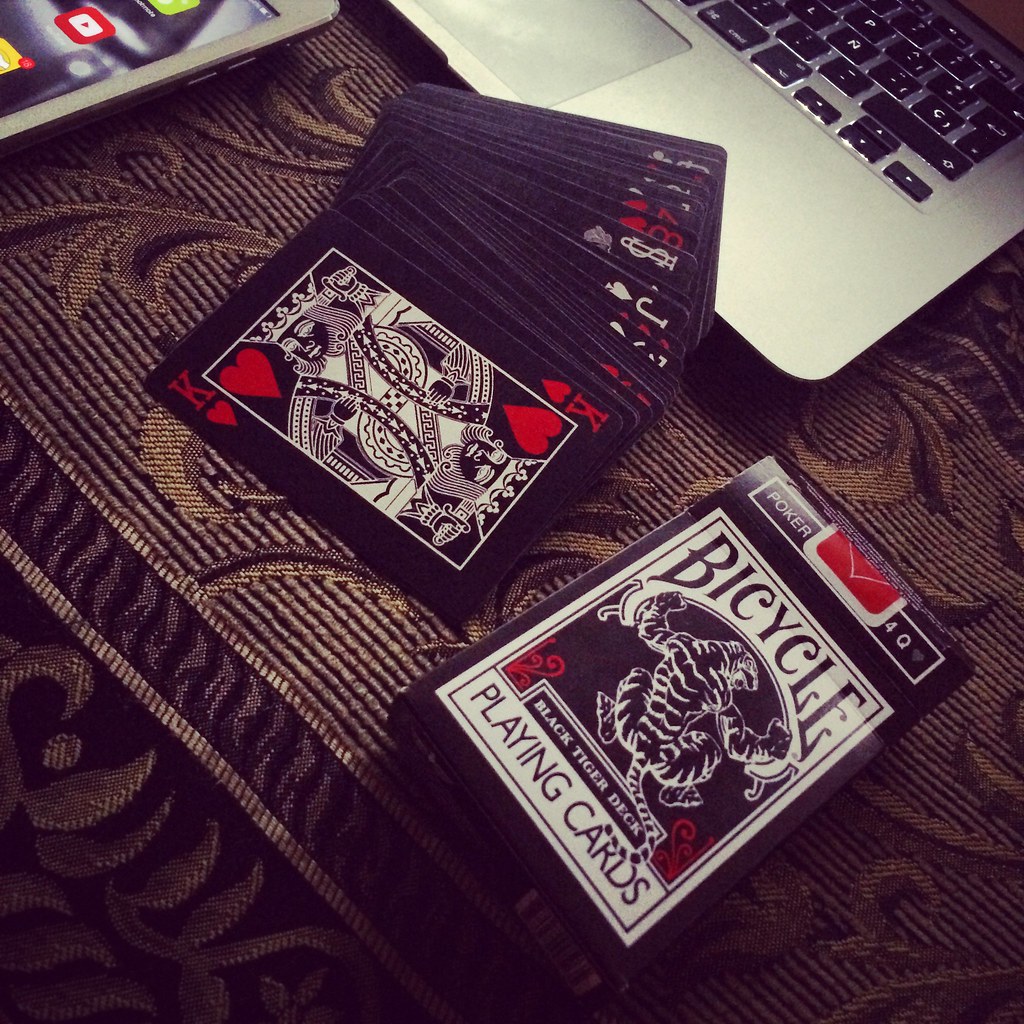A meticulously structured scene showcases a black deck of Bicycle playing cards placed prominently in the foreground. The cards, housed in a sleek black box with white text and adorned with an enigmatic creature design, exude elegance. A few cards are creatively splayed out, partly on a textured tablecloth with an intricate design and partly on a gleaming MacBook Pro in the background, its illuminated Apple logo subtly glowing. An iPhone peeks from the upper left corner, adding a modern touch to the setup. The eye is drawn to the King of Hearts, accentuating the deck's striking black, white, and red coloration. The photograph captures a meta moment, with the scene reflecting the observer’s digital involvement, creating a blend of classic and contemporary aesthetics.